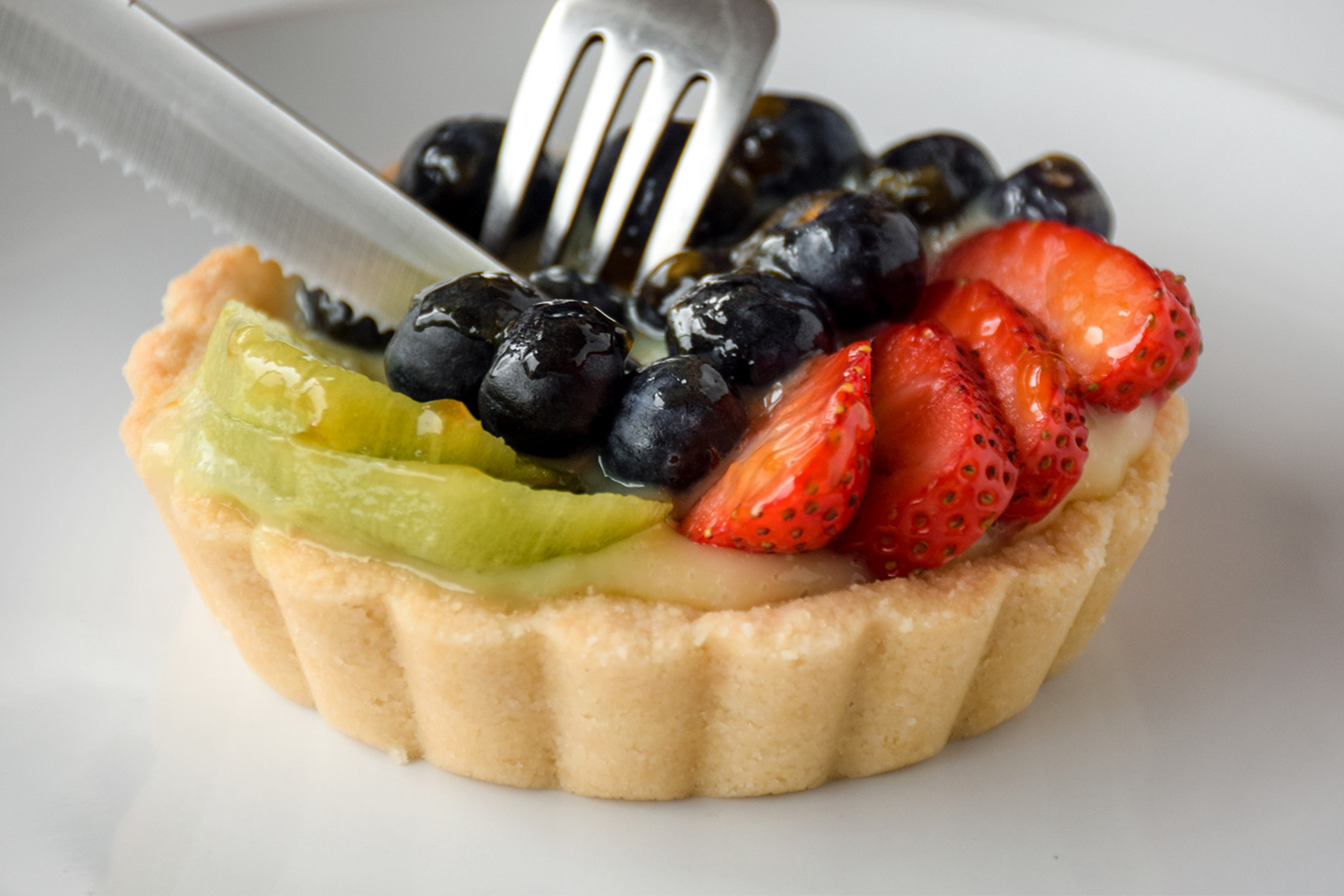This detailed photograph captures a delectable fruit tart brimming with a medley of vibrant fruits. The tart features an artfully arranged topping of succulent strawberries, delicate banana slices, vivid green kiwi, and plump blueberries, likely numbering around eight to ten. Positioned on a pristine white or whitish-gray plate, the scene captures the anticipation of indulgence as a knife and fork are poised to cut into the delicious treat. The serrated knife is actively engaged in slicing through the tart while the fork is angled backward, ready to assist in taking the first bite. The setting suggests the possibility of this being served at brunch or as a delightful dessert. The image vividly conveys the scene of someone about to enjoy this enticing fruit tart, highlighting its fresh, colorful presentation.